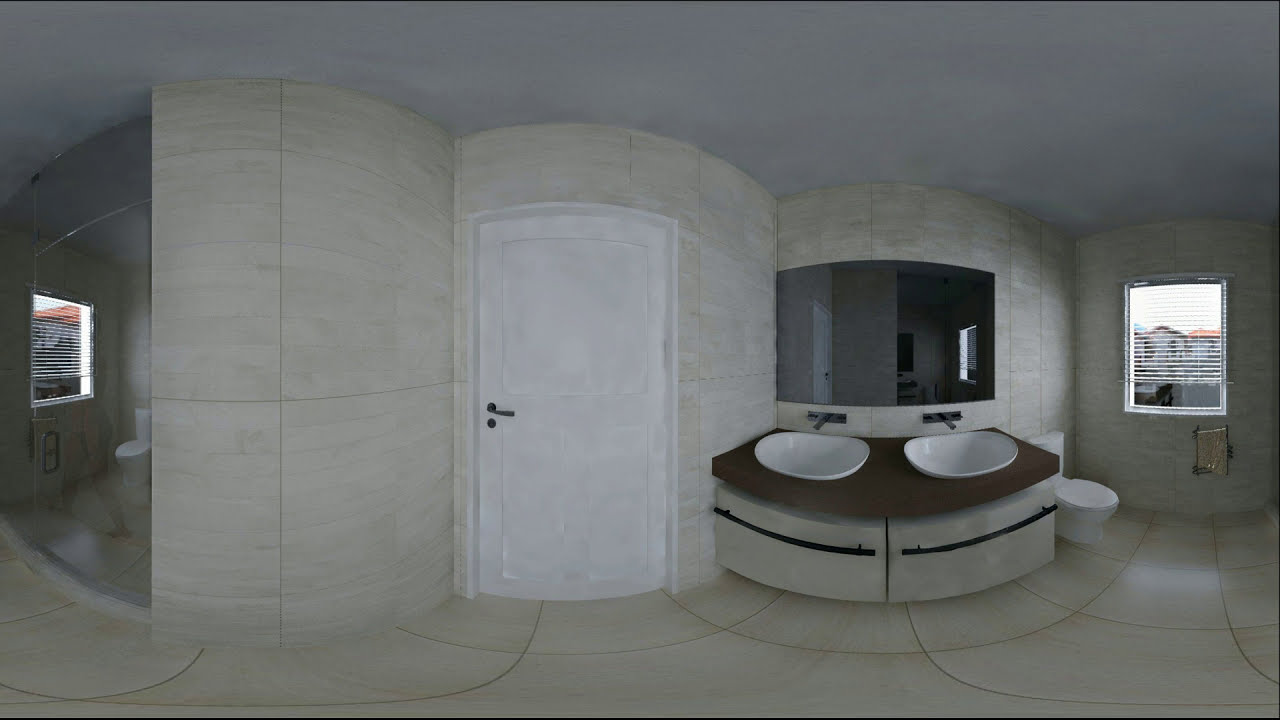The image depicts a spacious, sophisticated bathroom with a cohesive stone cream color scheme, encompassing the walls, ceiling, and floors, which all share a smooth, soft texture. The left-hand side features a wall of mirrors and a sleek, stone-colored panel. In the center, there is a pristine white door accented by a black handle. The right side of the bathroom showcases a double vanity with brown and cream tones, topped with two rectangular mirrors. Below the mirrors, the vanity houses two sinks, each with stylish fixtures. To the right of the sink area, a toilet is situated next to a small window with white blinds, offering views of neighboring houses, hinting at an apartment setting. Additionally, the bathroom includes a stand-up shower with minimal accoutrements, reflecting a high-end, possibly commercial design. The bright, natural daytime lighting enhances the clarity and the elegant ambiance of the space.